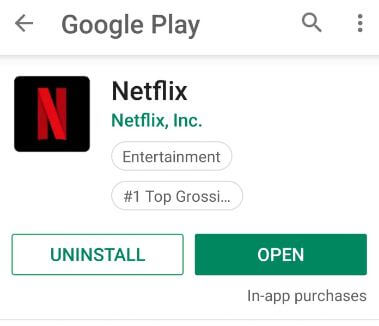Screenshot of a Google Play app page for Netflix. At the very top, on a black background, it reads "Google Play" with a left-pointing arrow on the left and a magnifying glass search icon followed by three vertical menu dots on the right. Below this navigation bar, the Netflix logo is prominently displayed: a black box with a red "N" next to the word "Netflix" in black text. Directly underneath, the text "Netflix, Inc." appears in teal. The background of the layout is white, giving a clean appearance. "Entertainment" is mentioned twice, indicating the app's category, and a partially visible label denotes "number one top grossing." Below this, two buttons are present: an outlined white box with teal green trim that says "Uninstall" in teal green, and a solid teal green box with white text that says "Open."